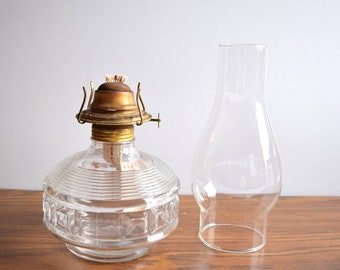The image features an old-fashioned, unlit glass lamp separated into two parts, positioned on a richly-colored, shiny wooden tabletop with a white wall in the background. The left part of the lamp, which serves as the base, is a transparent glass piece with a wider bottom. It includes a metal enclosure of gold color at its upper section, featuring a knob and thin protruding elements, resembling parts of a gas stove or a lamp connector. Visible within this section is a thin piece of white and red cloth, presumably serving as the wick. The right part of the lamp is a distinct, transparent glass cover with a cylindrical shape that bulges into a teardrop form. This piece is designed to fit onto the base, encapsulating the wick to complete the traditional lamp structure.